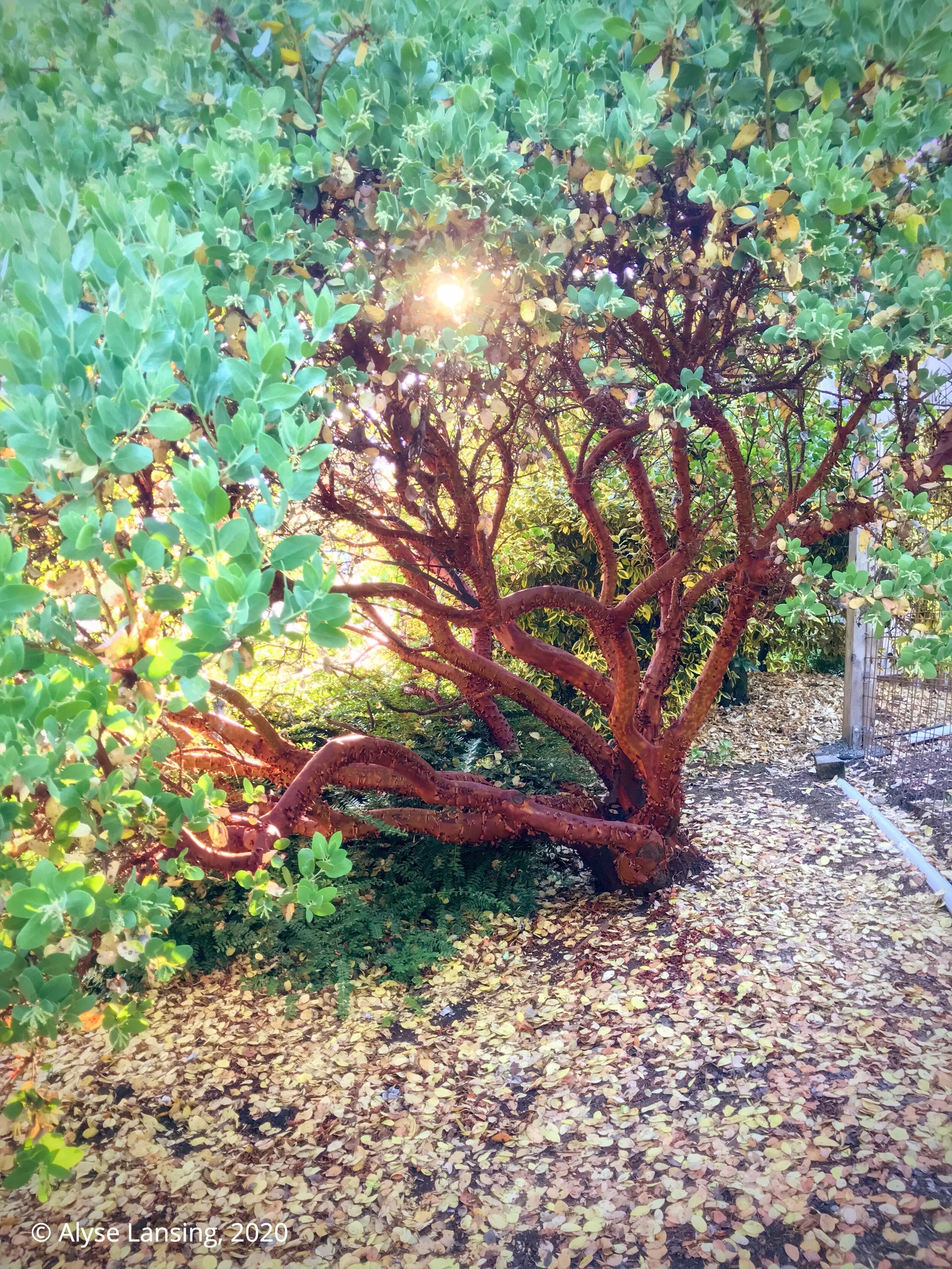This detailed edited photograph by Alyse Lansing, copyright 2020, captures a daytime scene of a tree with a dynamic, wind-swept appearance. The ground is an intricate carpet of light yellow and brown leaves, effectively obscuring the dirt beneath. The tree itself, starting in the middle of the photograph, has a stout trunk that quickly branches out into two or three thick, reddish-brown limbs. These limbs curve gracefully and support a dense canopy of small, soft, semicircular green leaves that fill the entire upper half of the image. The bright sunlight streams through the foliage, casting a warm yellow glow on the branches and illuminating the leaves, particularly on the top left side of the photograph. There may be a faint outline of a fence to the right, hinting at a landscaped setting. The image evokes the sense of early fall, with its rich play of light and textures and evokes a feeling of a peaceful natural space.